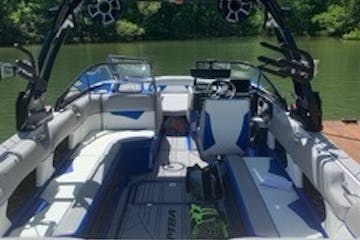The photograph depicts a modern, brand-new fishing boat moored at a dock on a greenish lake, surrounded by trees. The boat features a sleek design, adorned with white vinyl seats accented by patches of blue, which add a touch of color and style. The driver's seat and black steering wheel are positioned on the right side, with a passenger seat next to it on the left. Rising above the center of the boat is a distinctive black scaffolding, creating an arch and providing structural support. The deck of the boat is predominantly white, contributing to its clean and contemporary appearance. Despite the image’s low resolution, you can discern the wooden dock to which the boat is tied, suggesting it’s ready for an outing on the lake, ideally suited for fishing or leisurely exploration.